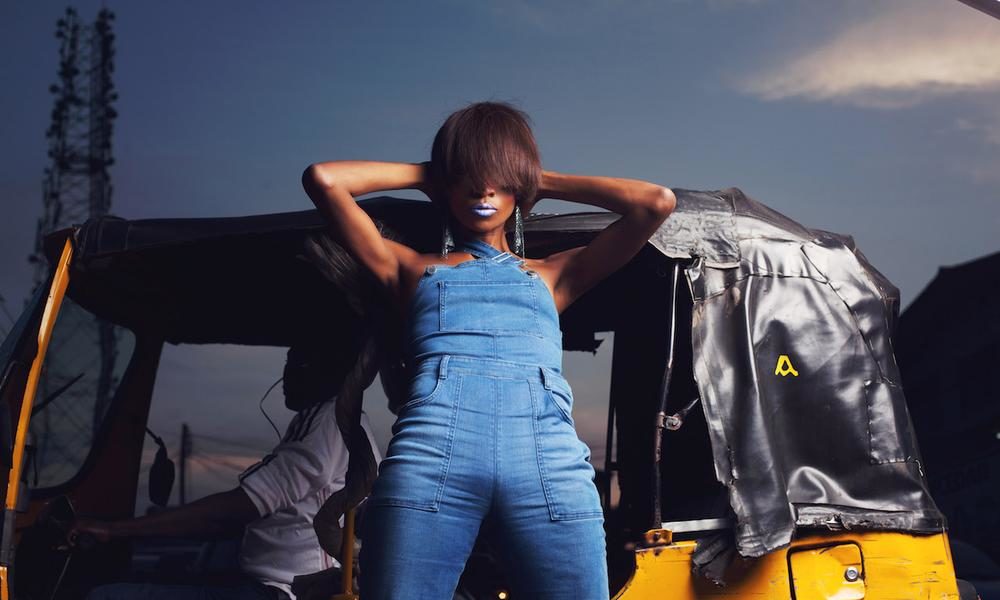The image is a detailed, color photograph in landscape orientation featuring a woman of African descent at its center. She has long, straight brown hair combed forward to completely cover her eyes, revealing only her nose and striking metallic blue lipstick. She is wearing tight, form-fitting blue jean overalls that crisscross at the neck, exposing her shoulders and giving the appearance of a halter top, with no shirt underneath. Her arms are folded behind her head, accentuating her pose with her elbows out to either side and her legs slightly spread. 

The woman is leaning back against a bright yellow vehicle, likely a rickshaw or Jeep, which has a black soft top. The vehicle is shown in profile, with a driver in a white shirt visible in the open cab. The background features a dark blue sky, suggesting either nighttime or twilight, with a metal tower, potentially an electrical or light tower, visible to the left side of the image. The overall style of the photograph leans towards photographic realism with elements of fashion photography.